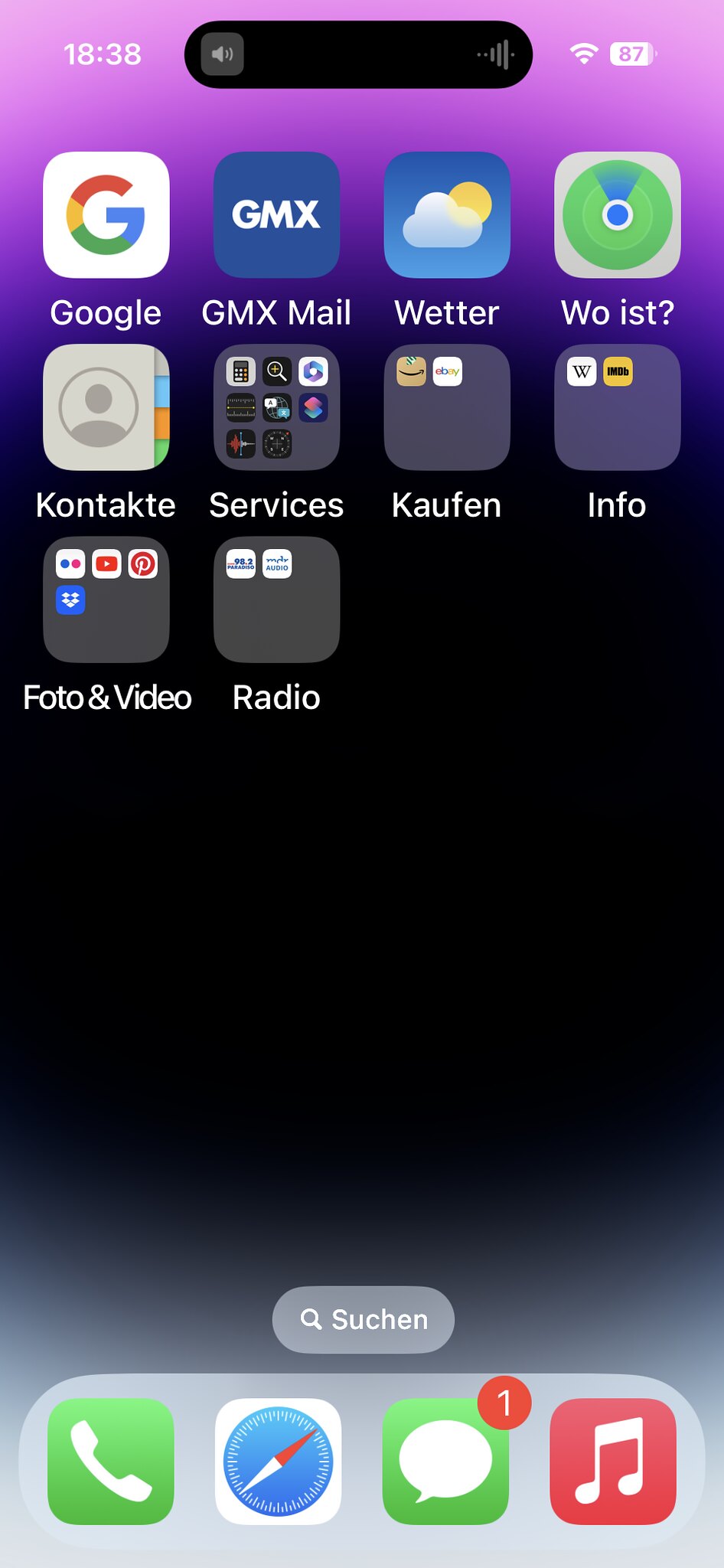The provided image is a landscape mode screenshot of a smartphone home screen.

The background is a light purple gradient transitioning from the top left corner to the upper right-hand corner. In the top left-hand corner, the time "18:38" is displayed, while the battery percentage "87%" is shown in the top right-hand corner.

The main section of the screen contains four columns and three rows of application icons:

1. **First Row:**
    - **Google**: The classic "Google" icon, labeled "Google."
    - **GMX Mail**: An icon labeled "GMX Mail."
    - **Weather**: A light blue icon featuring a translucent cloud with a sun in the upper right corner, labeled "Wetter."
    - **WOIST?**: A green icon with concentric circles in varying shades of green and white, with blue rays emanating from the center, labeled "WOIST?"

2. **Second Row:**
    - **Kontakte**: An icon resembling a notebook with a circle person icon over a half circle and four colored tabs—gray, light blue, orange, and green—labeled "Kontakte."
    - **Services**: A folder icon containing eight mini-icons, labeled "Services."
    - **Kaufen**: A folder icon with recognizable icons for Amazon and eBay inside, labeled "Kaufen."
    - **Info**: A folder icon containing "Wikipedia" and IMDb apps, labeled "Info."

3. **Third Row:**
    - **Foto & Video**: A folder icon with four mini-icons inside, including YouTube and Pinterest, labeled "Foto & Video."
    - **Radio**: A folder labeled "Radio," containing icons labeled "98.2" and "Audio."

At the bottom of the screenshot, there's a stationary dock with four icons:
1. **Phone**: A light green icon for phone calls.
2. **Compass**: A light blue icon with a compass.
3. **Messages**: A light green icon with a white speech bubble, marked with a "1" notification indicator.
4. **Music**: A red icon with white music notes.

This detailed structure offers a comprehensive view of the smartphone's home screen layout, providing clear identification and descriptions of each icon and folder.